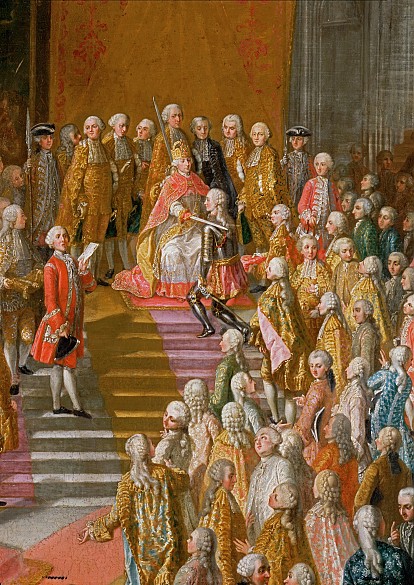The painting from the late 18th century vividly depicts a grand knighting ceremony, likely set in England. Central to the scene is a king, distinguished by his crown, flowing gown, and richly adorned red cape, seated at the apex of a set of stairs. He is in the act of knighting a gentleman clad in full armor with a powdered white wig, who kneels reverently before him, the king's sword touching his left shoulder. The backdrop is dominated by an expansive yellow wall interspersed with elements of red, adding to the regal atmosphere.

Surrounding the central figures is a diverse assembly of nobility, characterized by the period's formal attire. The men are prominently dressed in breeches, white tights, and pointed shoes, their outfits further embellished by tricorn hats and the flowing, stylized coats in hues of gold, blue, and red. They all sport the iconic white powdered wigs indicative of the era. While the crowd is predominantly male, there are subtle indications of possible female presences, their attire blending with the men's opulent garb.

To the right, a notable cluster of these noblemen engage in various distractions—some converse animatedly, others gaze around, and few focus intently on the ceremony. Behind the king, more members of the court, both men, and presumed women in capes, stand as part of the audience, contributing to the painting's rich tapestry of social hierarchy and courtly splendor.